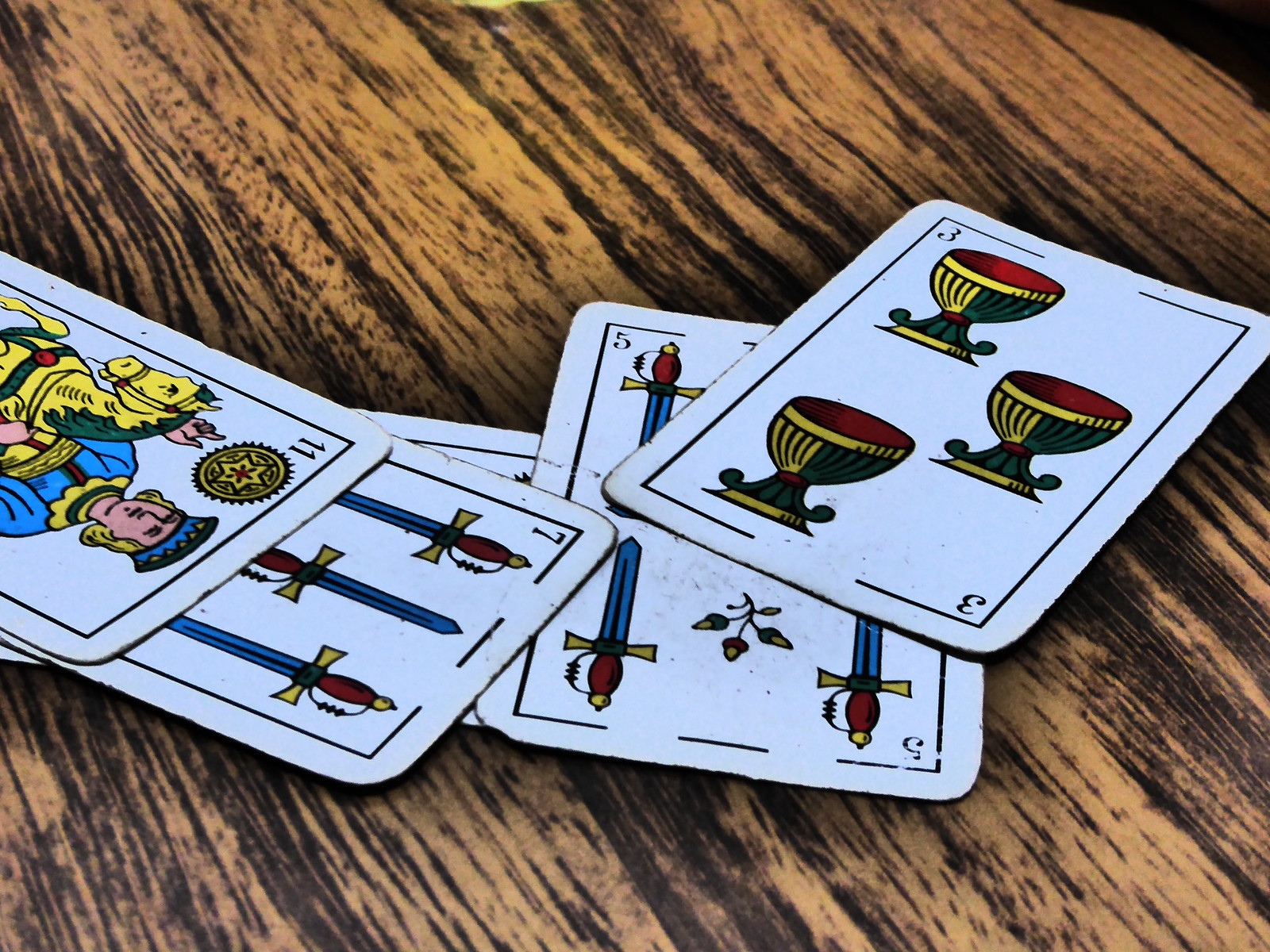This image showcases a set of five playing cards laid out on a weathered, wooden table. The table, occupying nearly the entire background, features a rich grain pattern with light yellow tones and dark veins that can only come from years of use. The grain runs diagonally from the top left to the bottom at an approximate 15 to 20-degree angle, adding depth and character to the scene. 

Just a small portion in the top right corner of the image is pitch black, breaking the monotony of the wooden texture. 

Spread across the center of the table are five playing cards. Four cards are face-up, revealing their distinct numbers in an unidentified card game with numerals instead of traditional suits. From left to right, the cards are as follows:

1. The first card is an 11.
2. The second card, a 7, is partially obscured by the 11.
3. The third card is hidden behind the 7, making its identity unknown.
4. The fourth card, a 5, is lightly covered at the top right corner by the adjacent card.
5. The fifth card is a fully visible 3, placed towards the top right of the image, just barely touching the right edge.

The arrangement and slight overlapping of the cards create a sense of casual disarray, enhancing the rustic atmosphere exuded by the worn table.